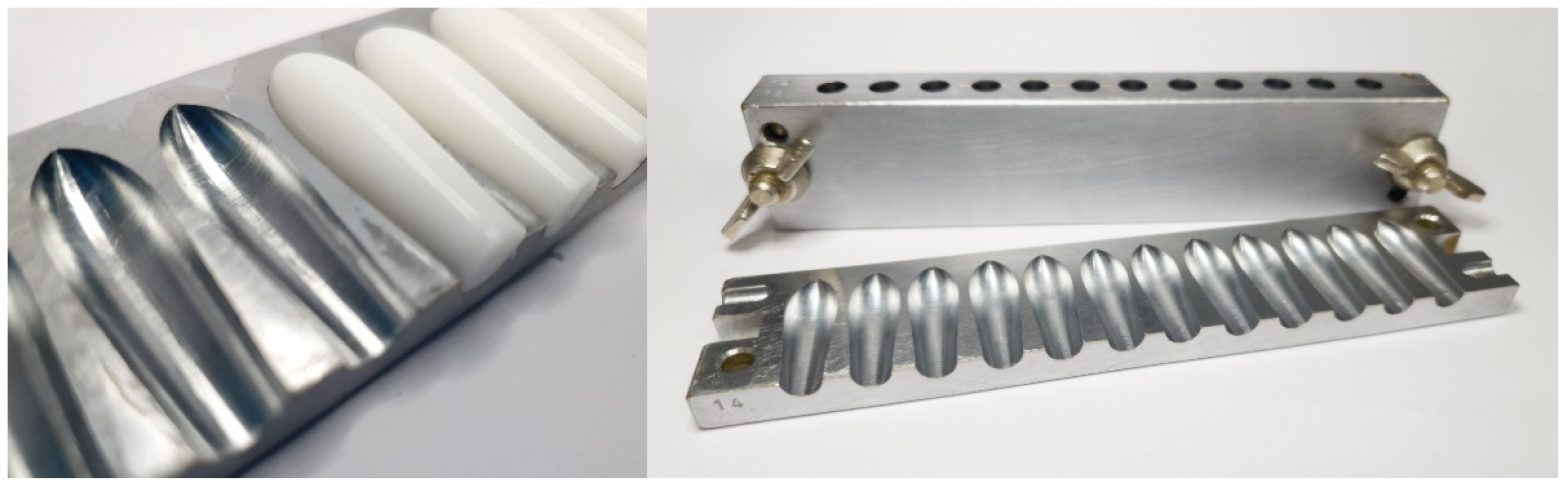This photograph combines two separate images to showcase a metal mold designed for creating cylindrical objects with ovoid tips, resembling either lipstick or suppositories. The left-hand side features a close-up highlighting the precise mold shape and the finished, white waxy products. The molds are silver and metal, with a surface showing numbered sections from 1 to 4, indicating the alignment for assembly. The detailed image on the right shows the entire mold setup in a more extensive view, displaying the two-part mold system. One half of the mold lies flat while the other half is propped up, revealing wing-nut bolts used for securing the mold pieces together. The full assembly of the mold shows holes at the top, where the liquid substance or metal is poured to create the final product. The contrasting backgrounds—darker gray on the left and white on the right—further highlight the different perspectives and details of the mold.